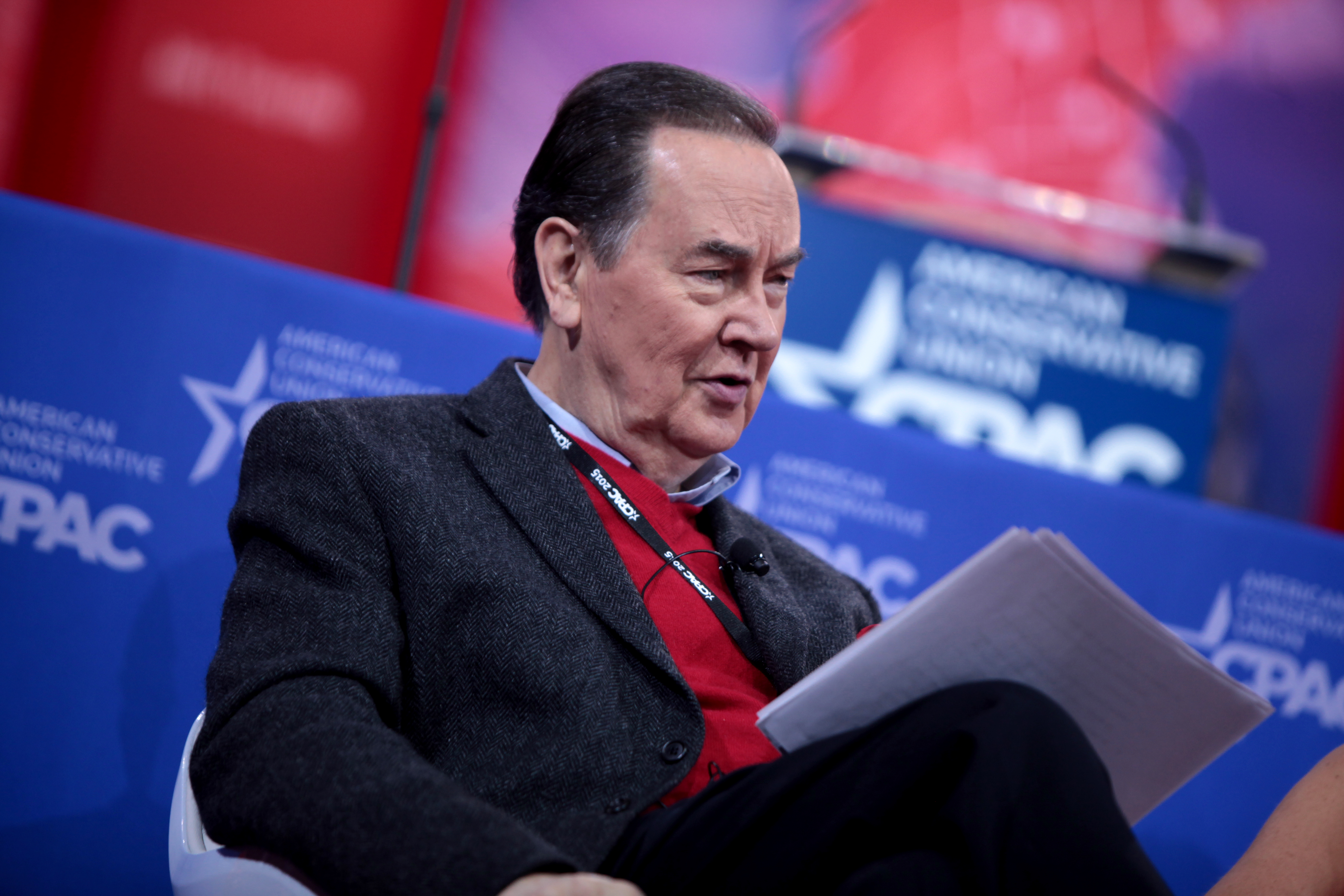The image features an elderly gentleman seated at the center, presumably participating in a political event organized by the Conservative Political Action Conference (CPAC). He is dressed in a dark gray suit jacket over a red shirt, with a hint of a blue collar peeking through. The man has dark hair, graying around his ears, and he wears a black lanyard printed with red text around his neck. His neutral expression suggests he is attentively listening to someone off-camera. He sits in a white chair with his legs crossed and a stack of white papers resting on his lap. The backdrop behind him prominently displays repeating CPAC logos against a blue background, along with text indicating "American Conservative Union." A blue and red stage setup is visible, featuring a screen and podium adorned with similar CPAC branding. The man's gaze is directed towards the right side of the image, where part of an unidentified person is partially visible, suggesting he may be seated next to someone.